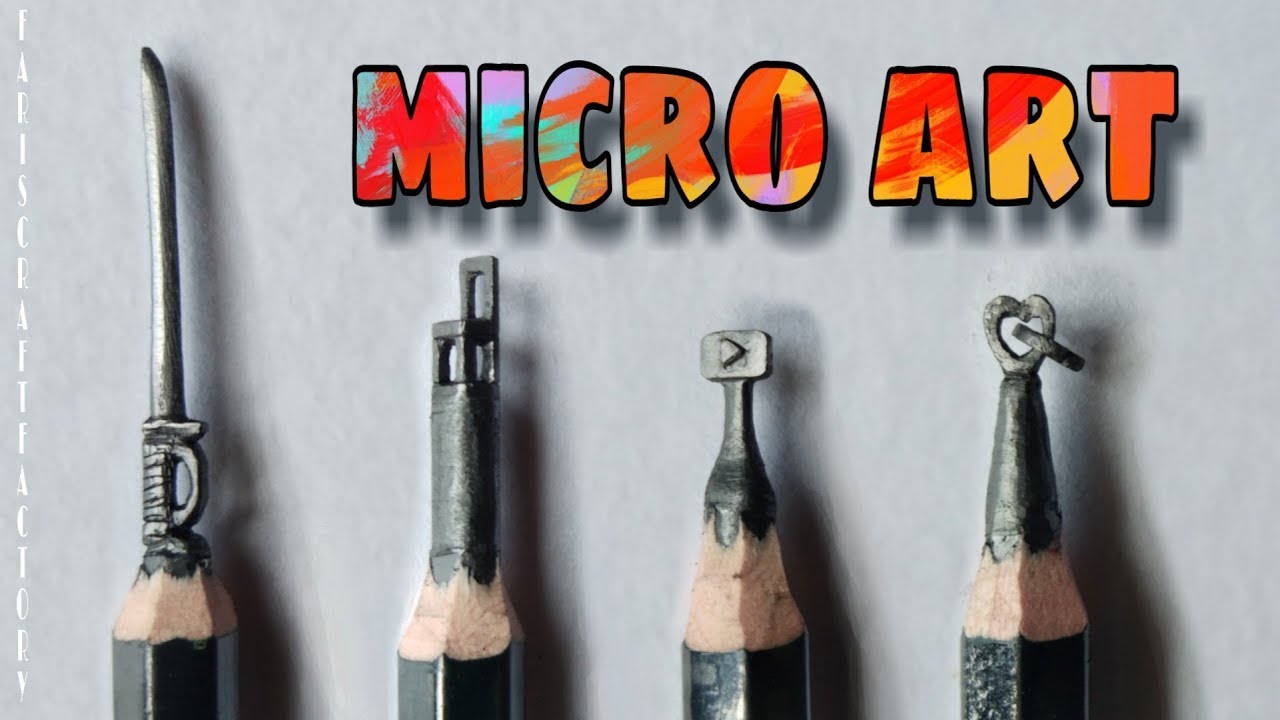This is a detailed close-up color photograph in landscape orientation featuring the intricately carved tips of four artist pencils. The pale gray background prominently displays multicolored text at the top that reads "Micro Art." Along the far left edge in vertically arranged white text, it says "Ferris Craft Factory."

The main focus is the four pencils, each carefully sharpened and transformed into miniature sculptures. Starting from the left, the first pencil's graphite has been masterfully carved into a detailed miniature sword with a long blade and ornate handle. The second pencil showcases an exquisitely crafted dining chair, complete with a high back and four legs. The third pencil replicates the YouTube play button, featuring a rounded rectangular shape with a small triangular play symbol in the center. The final pencil presents an open middle heart, intricately carved with another piece linking within it, resembling a chain. The pencils themselves are black, providing a stark contrast to the detailed carvings at their tips.